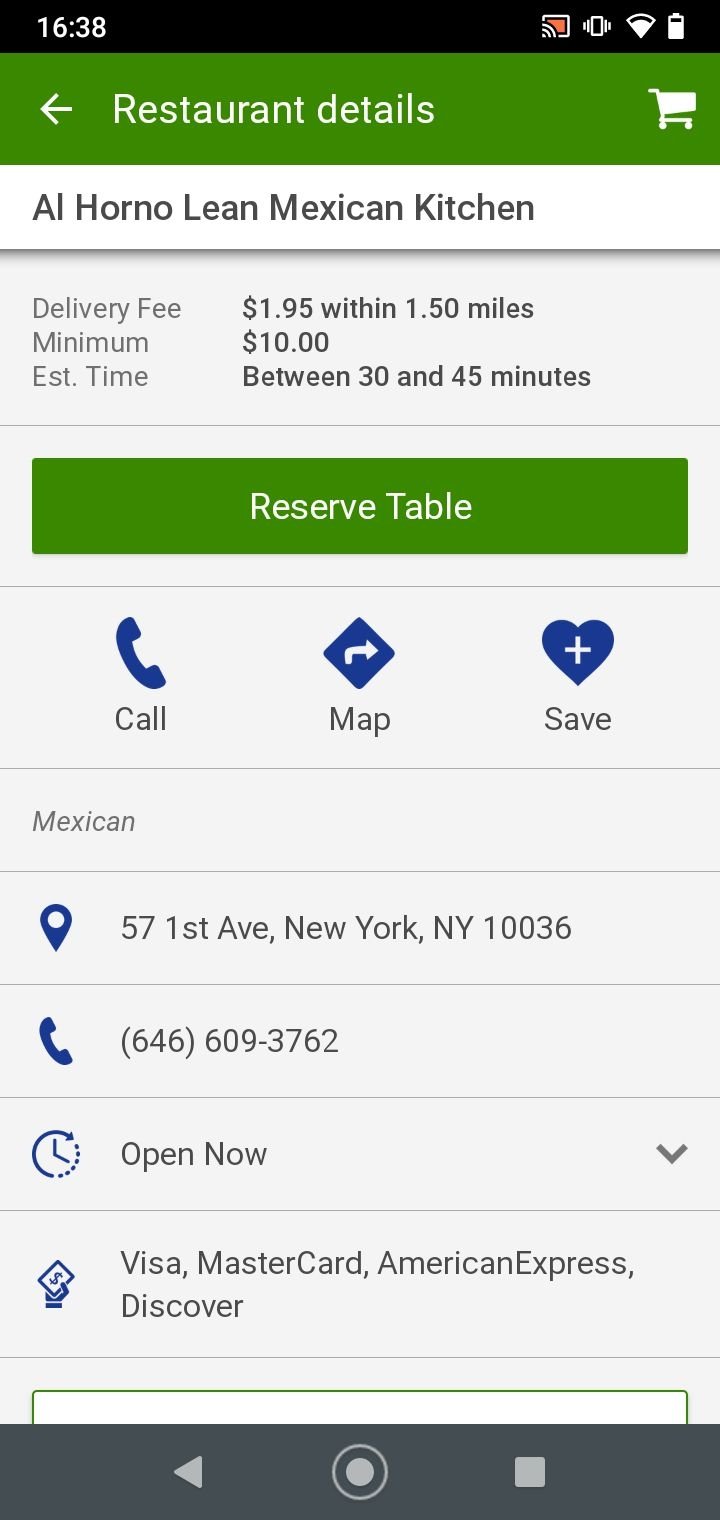This is a mobile screenshot depicting a detailed restaurant information page on a search app. The top bar is a vibrant green with the text "Restaurant Details" displayed in stretched, white letters that appear pixelated. Below this heading, the restaurant name "Al Horn Lean Mexican Kitchen" is written in prominent black letters.

Beneath the restaurant name, the layout is divided into two sections. On the left, categories such as "Delivery Fee," "Minimum," and "Estimated Time" are listed. Corresponding values for these categories are presented on the right side.

A large green bar dominates the area below, featuring the text "Reserve Table" in bold, white font. Under this, three icons are displayed: a telephone icon labeled "Call," a map icon, and a heart icon labeled "Save."

Additionally, the category "Mexican" is presented in gray font to the left. Further down, there's a vertical arrangement of icons beginning with a blue pin drop icon beside the address. A blue telephone icon is displayed next to the phone number, followed by a clock icon indicating the restaurant's status with the text "Open Now." Lastly, a paper icon with dollar signs is shown, detailing accepted payment methods, including Visa, MasterCard, American Express, and Discover.

At the very bottom of the screen, there's a black bar featuring navigation icons for home, back, and minimize.